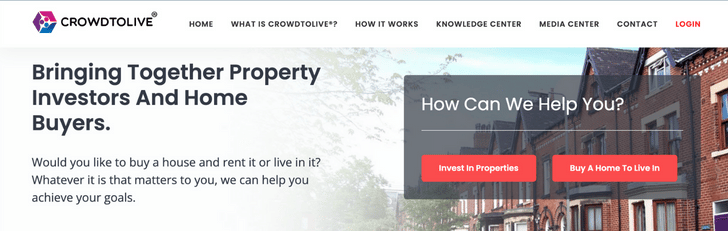At the top right of the image, there's a navigation menu. The first item says "Crowd to Live," followed by "Home" in black text, then "What is Crowd to Live?", "How it Works," "Knowledge Center," "Media Center," and "Contact." The final item on the menu is "Login" in red.

Below the menu, the background changes to gray. On the left-hand side, in black text, it says, "Bring together a property." Underneath that, the text continues with, "Investors and Home Buyers." There's a prompt stating, "Would you like to buy a house and rent it or live in it? Whatever it is that matters to you, we can help you achieve your goals."

An image of red brick townhomes is displayed, partially covered by a transparent black rectangle at the bottom. Inside the rectangle, in white text, it asks, "How can we help you?"

A thin white line separates sections of the page. At the bottom of the second section, there are two black rectangles. The first rectangle has "Invest in Properties" written in white capitalized text, and the next rectangle says, "Buy a Home to Live In," also in white.